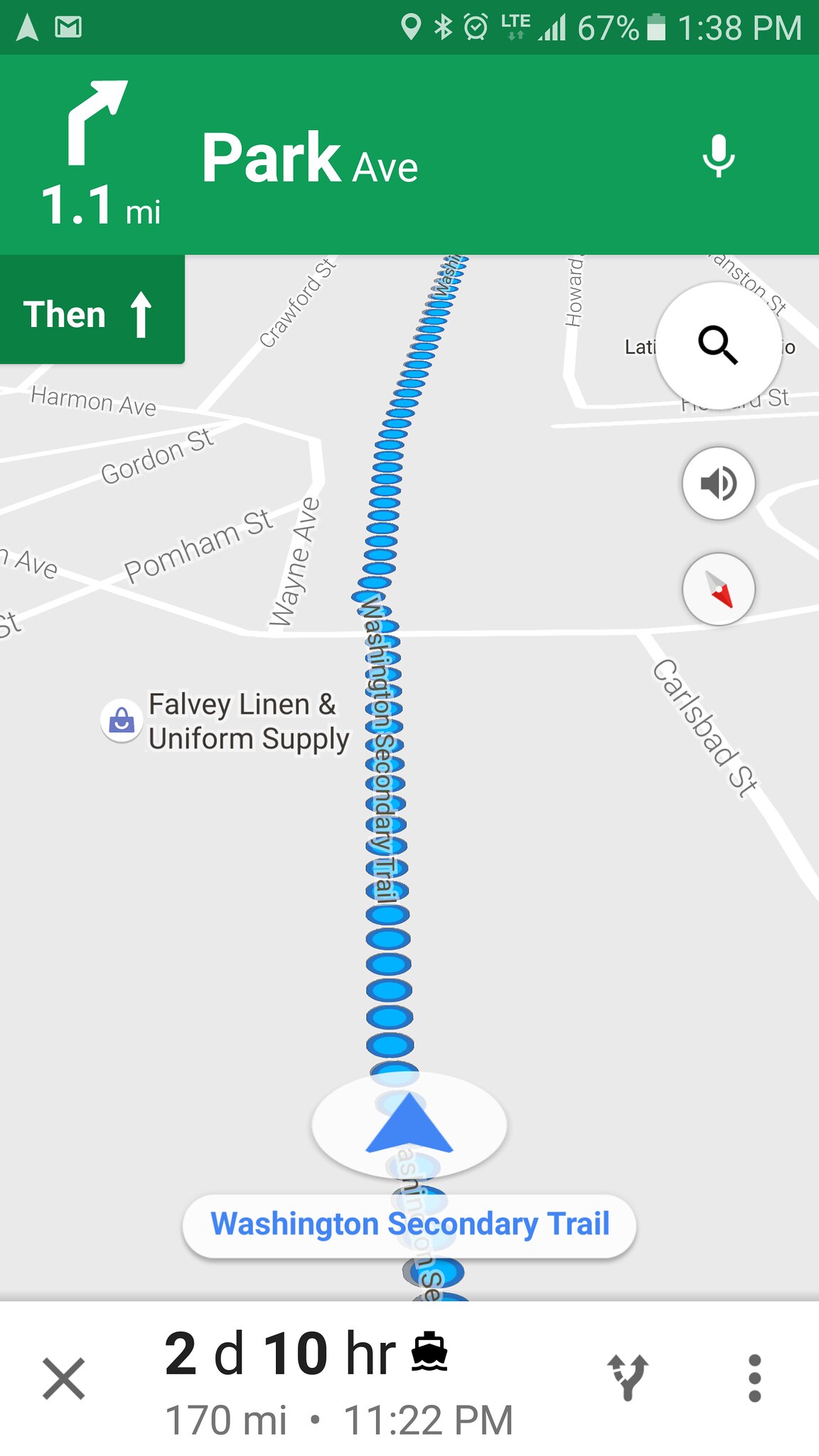This screenshot of a smartphone display features the Google Maps interface. Prominently, an arrow at the top directs diagonally to the right, indicating a distance of 1.1 miles to Park Avenue. Below this, the map reveals a detailed street layout with various marked streets and a prominent blue directional arrow pointing upward, marking the Washington Secondary Trail route. 

At the bottom of the map, a summary box states "two days, 10 hours, 170 miles," and the current time as "11:22 p.m." Above the map interface, the status bar of the smartphone is visible, showing icons for Google Maps, Bluetooth, an alarm clock, LTE network, and a battery level at 67%. The current time is displayed as 1:38 p.m.